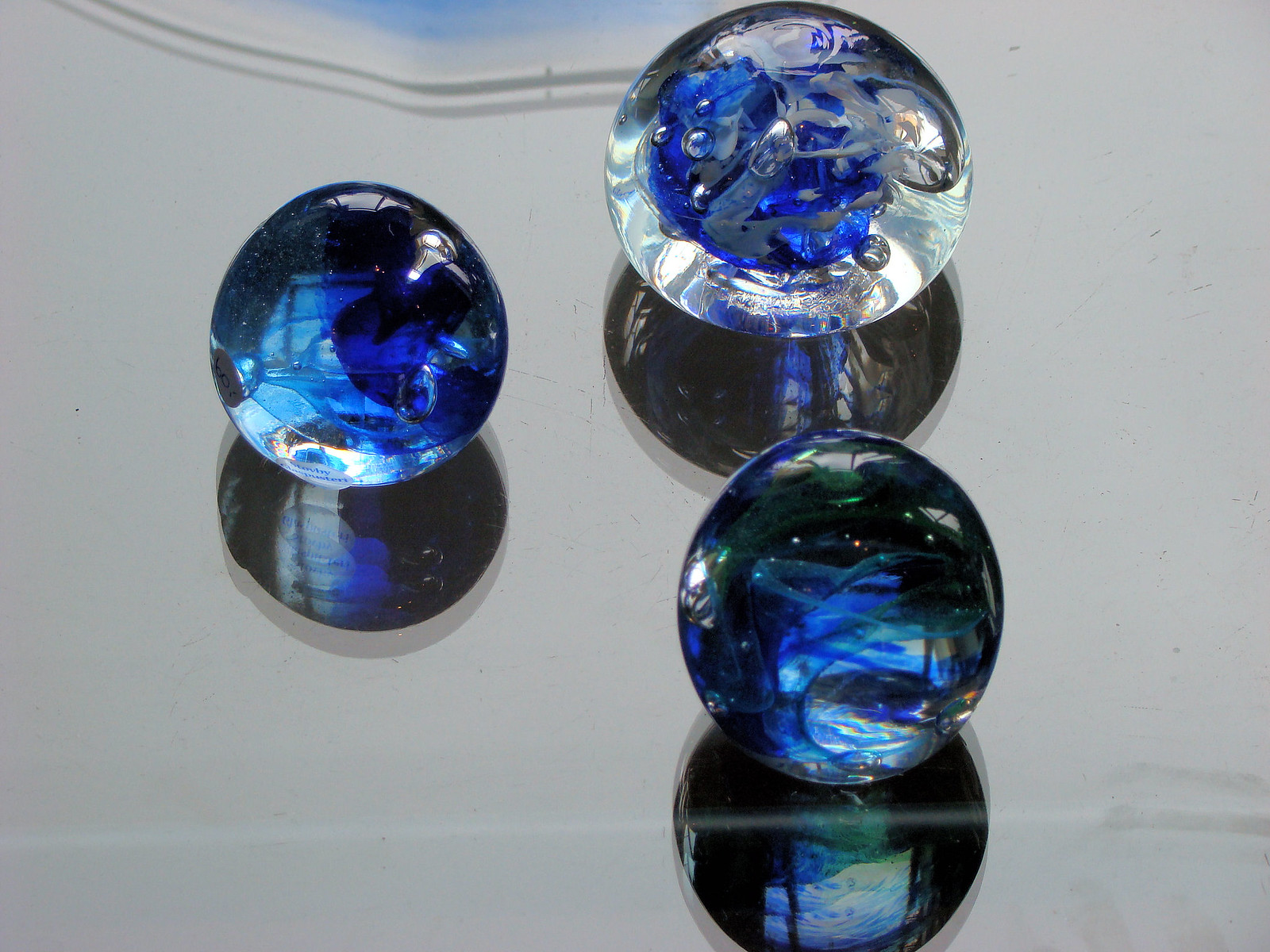The image is a close-up of three glass spheres, arranged in a triangular formation on a polished, pale grey mirrored surface. Each sphere, resembling a marble, is a beautiful mix of crystal clear and various shades of blue. The left sphere features swirling blue ink with clear liquid and visible bubbles, some appearing black. The right sphere contains a blue cloud along with grayish silver lines and clear bubbles, all within a larger clear sphere. The bottom sphere has dark blue liquid and darker areas, with the bottom portion being clearer than the top. Each sphere casts a shadow and reflects its colors onto the shiny surface.